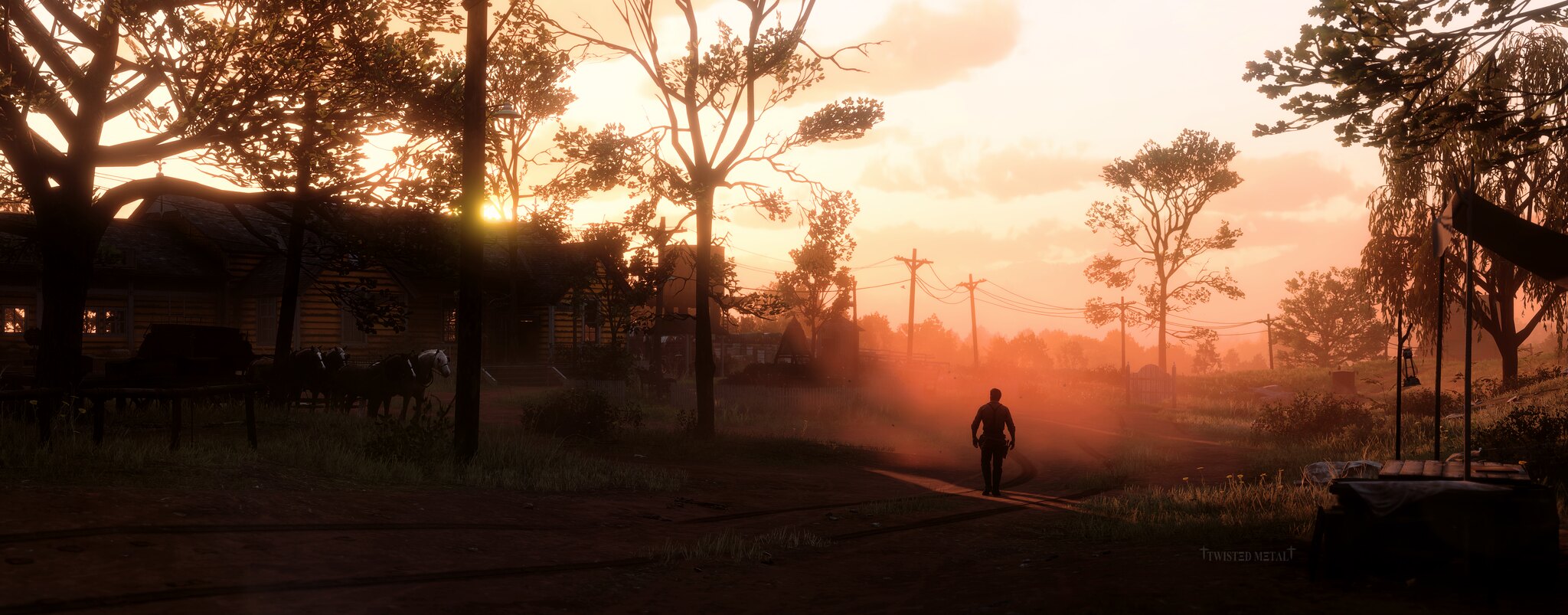The image appears to be a highly detailed digital artwork or game screenshot, possibly reminiscent of "Red Dead Redemption." It depicts a serene yet somewhat eerie rural scene during sunrise or sunset, casting a warm, orange-pink glow across the landscape. In the foreground, an individual, likely a man, is walking down a dusty path lined with trees. The silhouette of this lone figure is striking against the backdrop of shadowy trees on both the left and right sides. On the left, near the horizon, stands a one-story farmhouse with horses grazing in front. Further back, a series of five or six utility poles with power lines stretch across the sky, adding a touch of modernity to the rustic setting. The sky itself is a gradient of light yellow to pink, with wispy white clouds, enhancing the twilight atmosphere. The ground is grassy and hints of dust create an orangish tint, adding to the detailed composition of this tranquil yet haunting scene.